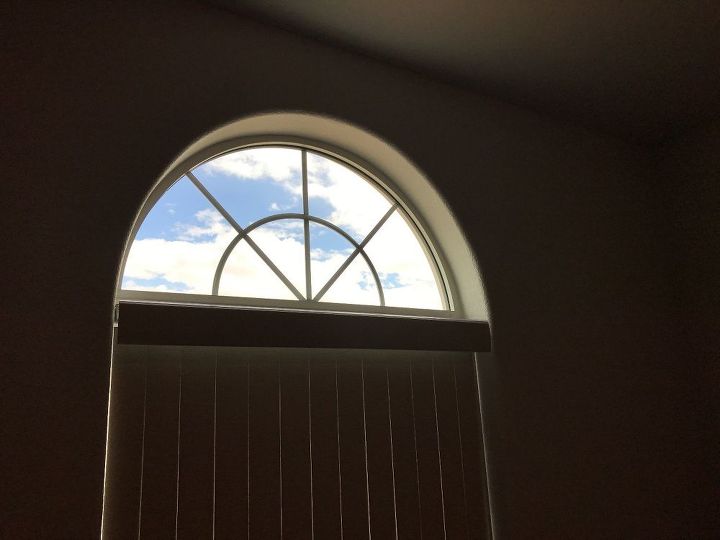This photograph captures the interior of a dimly lit room with a prominent arched window at its center. The window has a flat bottom and a semi-circular top, featuring several glass panels arranged to fit its unique shape. The bottom portion of the window is draped with curtains, allowing only slivers of light to filter through, while the top portion remains uncovered, offering a view of the outside sky. The external sky is a dark blue hue with thin, white and gray clouds scattered across it. The walls inside the room appear to be dark brown, possibly due to the lack of light, while the ceiling shows a slightly lighter spot towards the top. A distinct brown shadow line runs from the center of the wall down toward the right. The photograph evokes a sense of solitude, with the primary illumination coming from the daylight outside, subtly highlighting the architectural details of the semi-circular window.